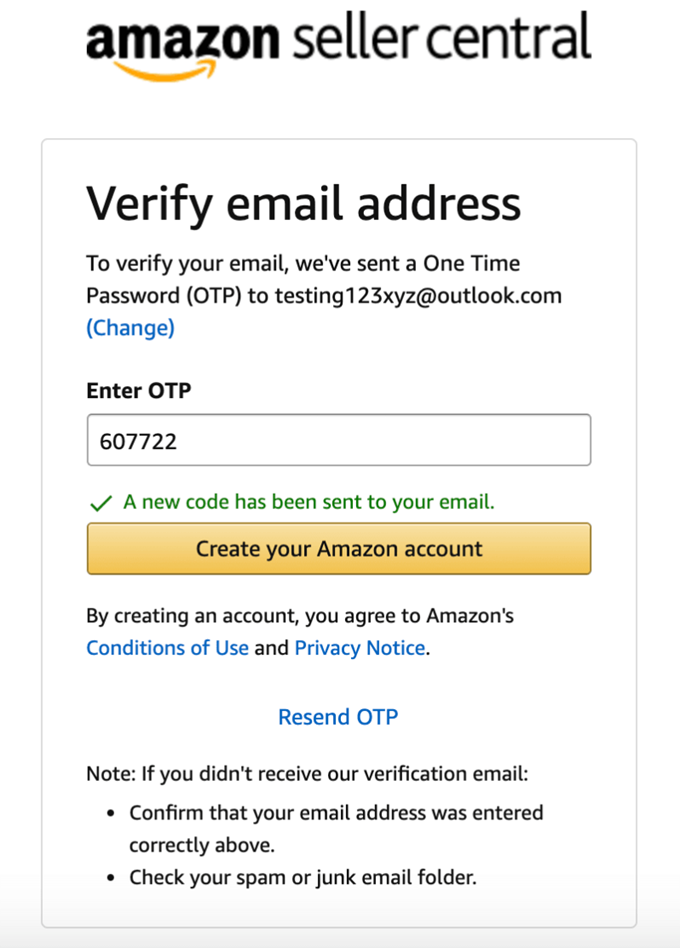The image displays a verification screen for Amazon Seller Central on a white background. At the top, in bold black letters, it reads "Amazon Seller Central," accompanied by the iconic orange curved arrow under the word "Amazon." Beneath this, a gray outlined box contains black text stating "Verify email address." 

Further down, the message indicates that to verify the email, a one-time password (OTP) has been sent to testing123xyz@outlook.com. To the left of this notification, the option to change the email address is highlighted in blue font.

Below, a grey outlined white input box contains the OTP "607-722" in black text. Underneath this box, a green check mark is displayed alongside a message in green text stating, "A new code has been sent to your email."

An orange button with black text, located below, invites users to "Create your Amazon account." A disclaimer follows, informing that by creating an account, users agree to Amazon's "Conditions of Use" and "Privacy Notice," with these terms highlighted in blue for emphasis.

The footer section includes a grey outlined note, reading "Resend OTP." Below this, another message in black text provides guidance: "Notice: If you didn't receive your verification email, confirm your email address was entered correctly above, and check your spam or junk email folder."